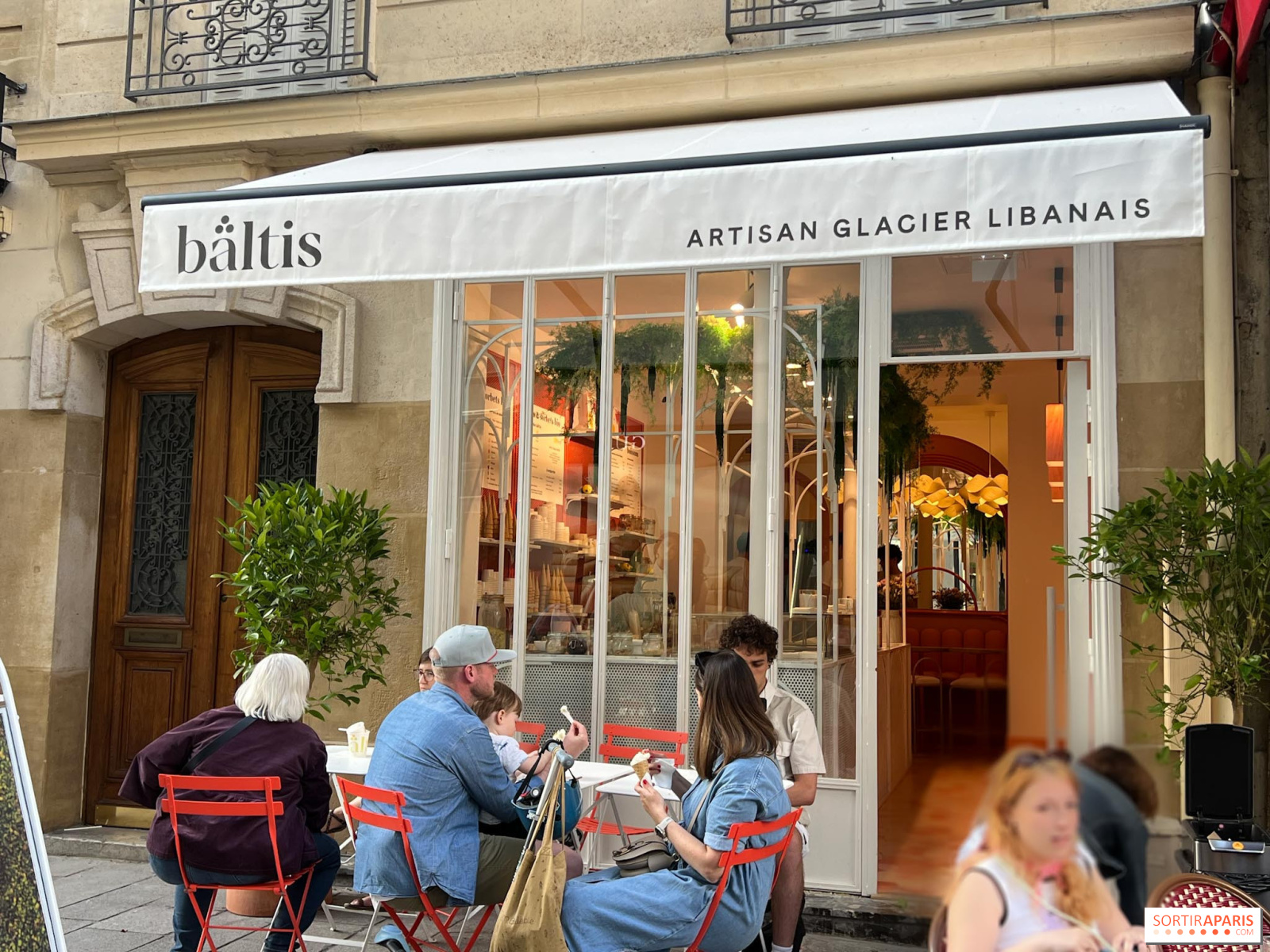The image shows a charming outdoor dining scene in front of a small cafe or restaurant, likely located in Paris, as suggested by the text "SORTIRA PARIS" in the lower right corner. The cafe is part of a multi-storied, light tan concrete building with two wrought iron-decorated balconies above. The establishment has a white canopy or awning extending from the top of its windows, inscribed with "BALTIS" in dark gray, with three dots above the "A". To the right of the name, it reads "ARTISAN GLACIER LIBANAIS" in all caps dark gray letters.

In front of the cafe are several white-bordered windows and double dark brown wooden doors with rectangular glass panes, one of which is open, allowing a glimpse inside. The outdoor seating area features tables draped in white tablecloths and surrounded by small redwood chairs. Various patrons, including families, men, women, and children, are casually sitting and enjoying their meals. There are also some decorative plants on either side of the windows, adding to the cozy and inviting atmosphere. The scene is set during the daytime, evidenced by the natural light, although the sky is not visible in the image.